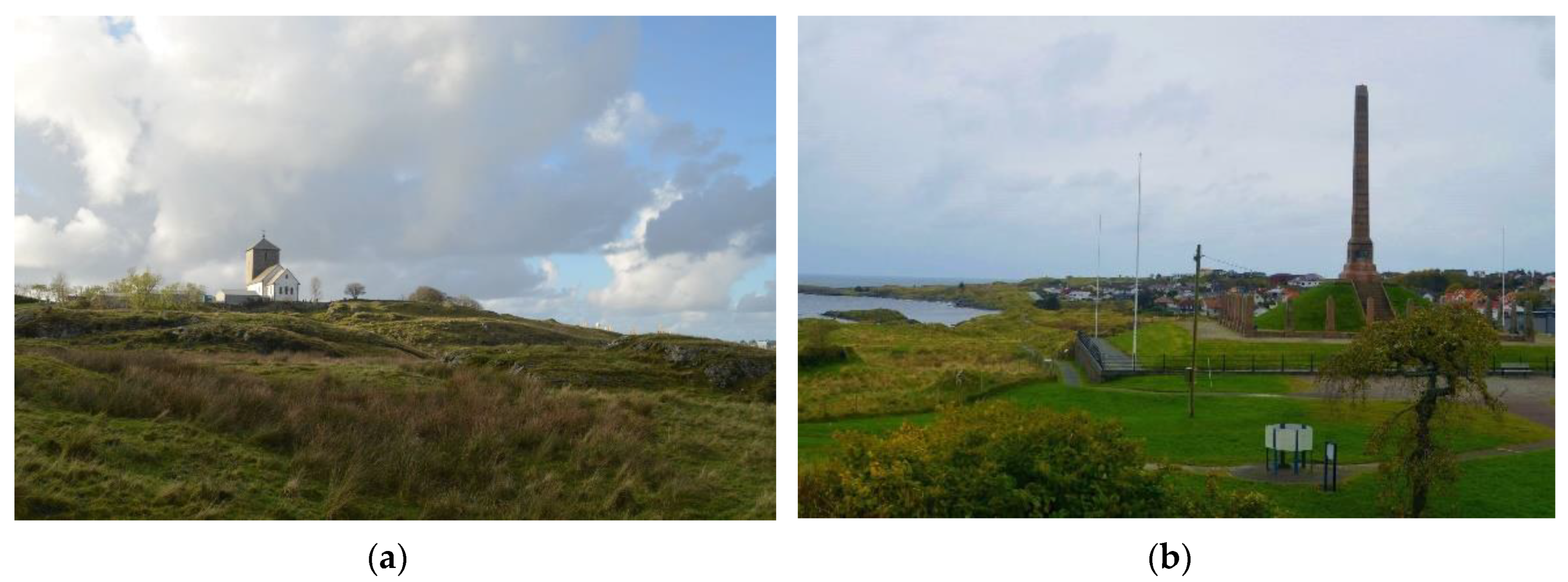This image is a collage of two outdoor photos labeled A on the left and B on the right. 

Photo A depicts a serene landscape with a vast, grassy field in the foreground. A small, white house, reminiscent of a church with a cathedral-like top and three visible windows, is situated on a hill in the far background. The sky occupies much of the scene, filled with blue hues and fluffy, white clouds. To the right of the house, a silo adds a touch of rural character to the landscape. The field itself is covered with green grass and patches of tall, brownish brush, enhancing the natural, tranquil ambiance of the setting.

In contrast, Photo B presents a more developed and varied landscape. The foreground features a mix of light and dark green grasses, interspersed with a dark gray pavement sidewalk. To the left, a light blue lake is surrounded by greenery, while scattered trees with lush green leaves dot the area. A prominent monument or tower rises from a small mound at the center, flanked by street lights and power lines. The background shows additional buildings, perhaps houses or cars, in muted tones of brown and white. The sky is similar to that in Photo A, with light blue hues and wisps of thin, white clouds indicating a slightly overcast day.

Overall, the images contrast a simpler, rural scene with a more complex, semi-urban setting, highlighting the subtle beauty of both locales.